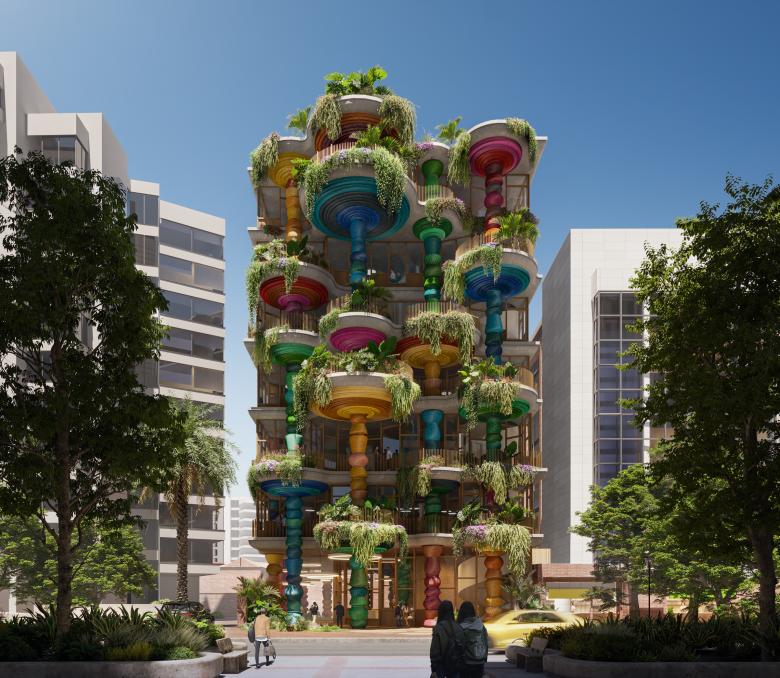In the bustling cityscape, the central focus is a striking, six-story tall building that stands out with its futuristic, tropical aesthetic. This unique structure, likely a major tourist attraction, features a series of balconies shaped like wine cups or martini glasses, supported by columns in vibrant hues of pink, blue, yellow, green, and red. These eye-catching balconies are adorned with lush vegetation, adding to its distinctive charm. Flanked by two sleek, modern white buildings, the colorful centerpiece captures all attention with its imaginative design.

The photograph captures a sunny day with a bright blue sky, adding to the vibrancy of the scene. Taken from across the street, the image includes a couple of trees on the far left and right edges and several people in the foreground, one approaching the building and others scattered nearby, emphasizing human interest and activity. A car is also visible driving past, integrating the scene seamlessly into the urban environment. The focus remains firmly on this exceptional building, whose unique look and prominent placement draw the eye and spark curiosity.